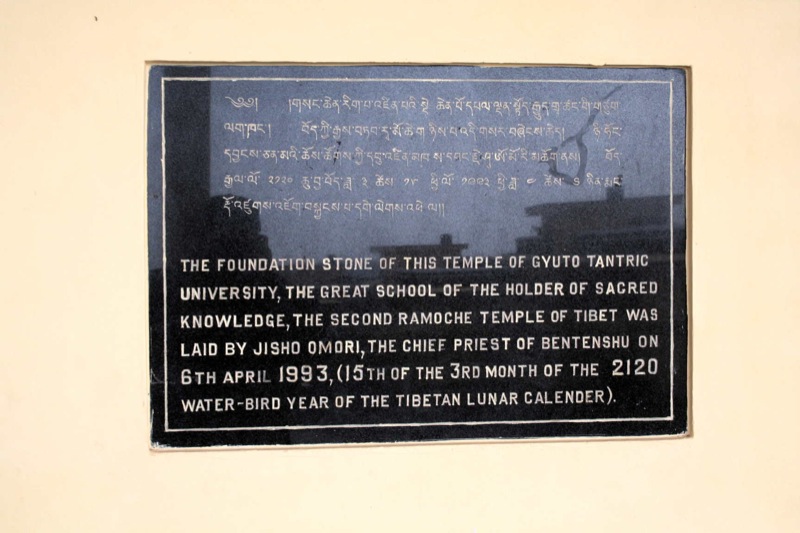The image depicts a black reflective marble placard set into a recess on a tan-colored painted wall, which appears beige in some descriptions. The placard features a delicate white line serving as a border. The top half of the placard has text etched in a Southeast Asian script, comprising five lines. Beneath this foreign text, the English inscription is detailed and reads: 

"The foundation stone of this temple of Gyūto Tantric University, the great school of the holder of sacred knowledge, the second Ramosh Temple of Tibet, was laid by Jisō Omori, the chief priest of Benten-shū, on 6th April 1993, 15th of the third month of the 2120 water bird year of the Tibetan lunar calendar.”

This plaque signifies an important historical moment, marking the founding of a significant religious and educational institution.